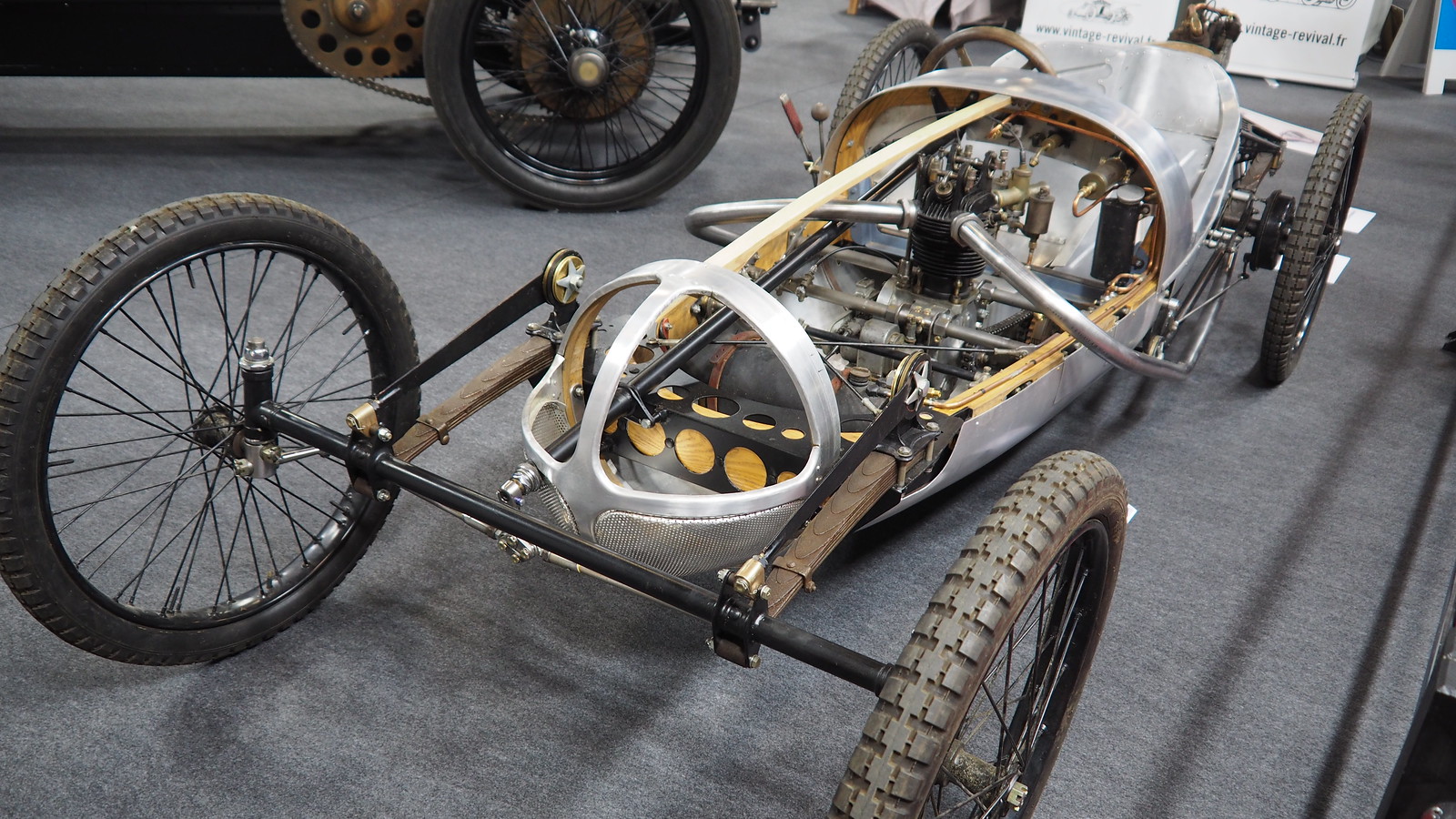The image is a horizontal rectangular photograph showcasing a homemade race car, seemingly improvised from various materials. The main body of the car is constructed from metal, featuring pipes that run along the sides and form part of the steering apparatus, connecting the front and back wheels—all of which resemble bicycle wheels. The car's axis spans the bottom, with the cockpit located just in front of it for the driver. The cockpit contains a black seat adorned with large yellow dots. Beneath the hood, a gas pedal is visible, and likely a brake component on the opposite side. The vehicle sits inside a garage, positioned slightly to the right and angled downward to the bottom left corner. Adjacent to it is another, larger vehicle with bigger tires and a visible brown gear near its left tire. Colors in the image range from silverish gray and black to birch, brown, and bright blue. The background features posters, suggesting a racing theme or environment. The overall setting indicates a workspace or garage, with an emphasis on homemade ingenuity and resourcefulness.